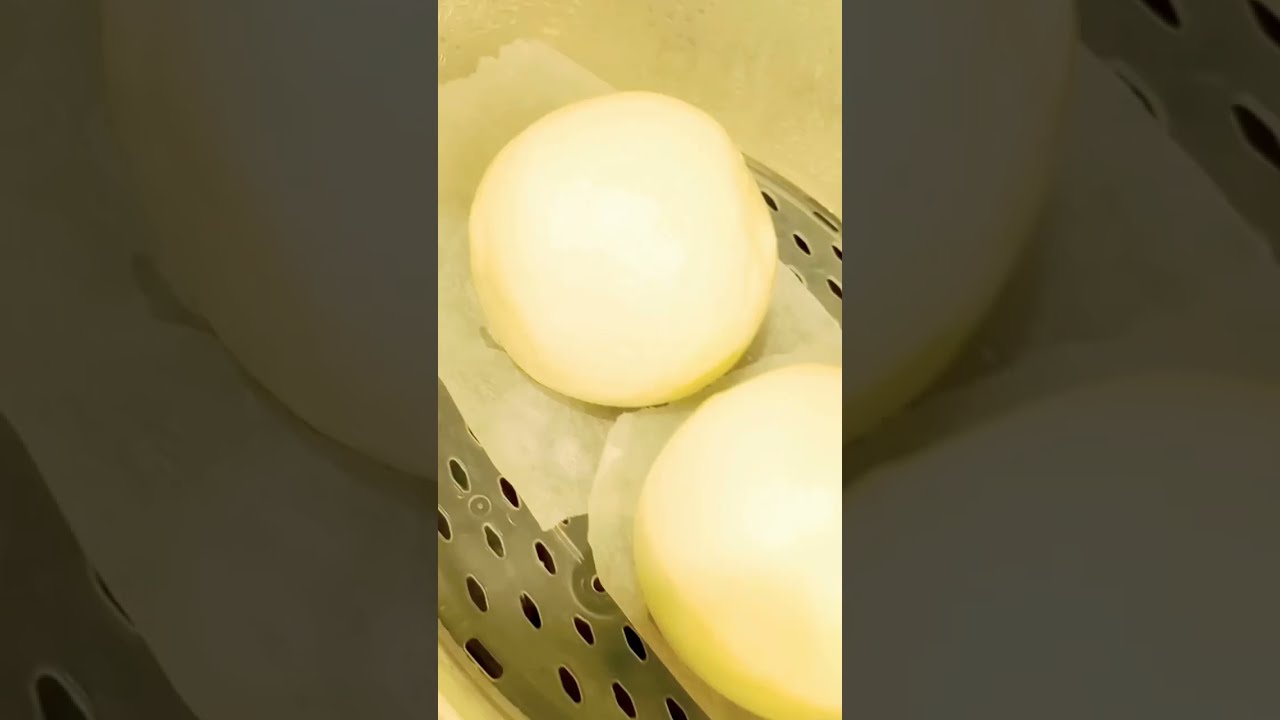The image captures a close-up view of two white spherical objects, potentially food items like dough balls or round vegetables, placed inside a kitchen container. The primary focus is on one spherical object in the center, with another partially visible ball emerging from the bottom-right corner. These objects rest on strips of wax paper, which lie on a plastic grid with oval-shaped holes. The vertical photo is centrally framed within a larger, horizontally oriented background of the same image, zoomed in and faded. The image captures a blend of colors including white, pale yellow, tan, and silver, with the overall hue being light and clear. The background of the photo appears to be a gray or off-white porcelain material, providing a clean and minimalist aesthetic.